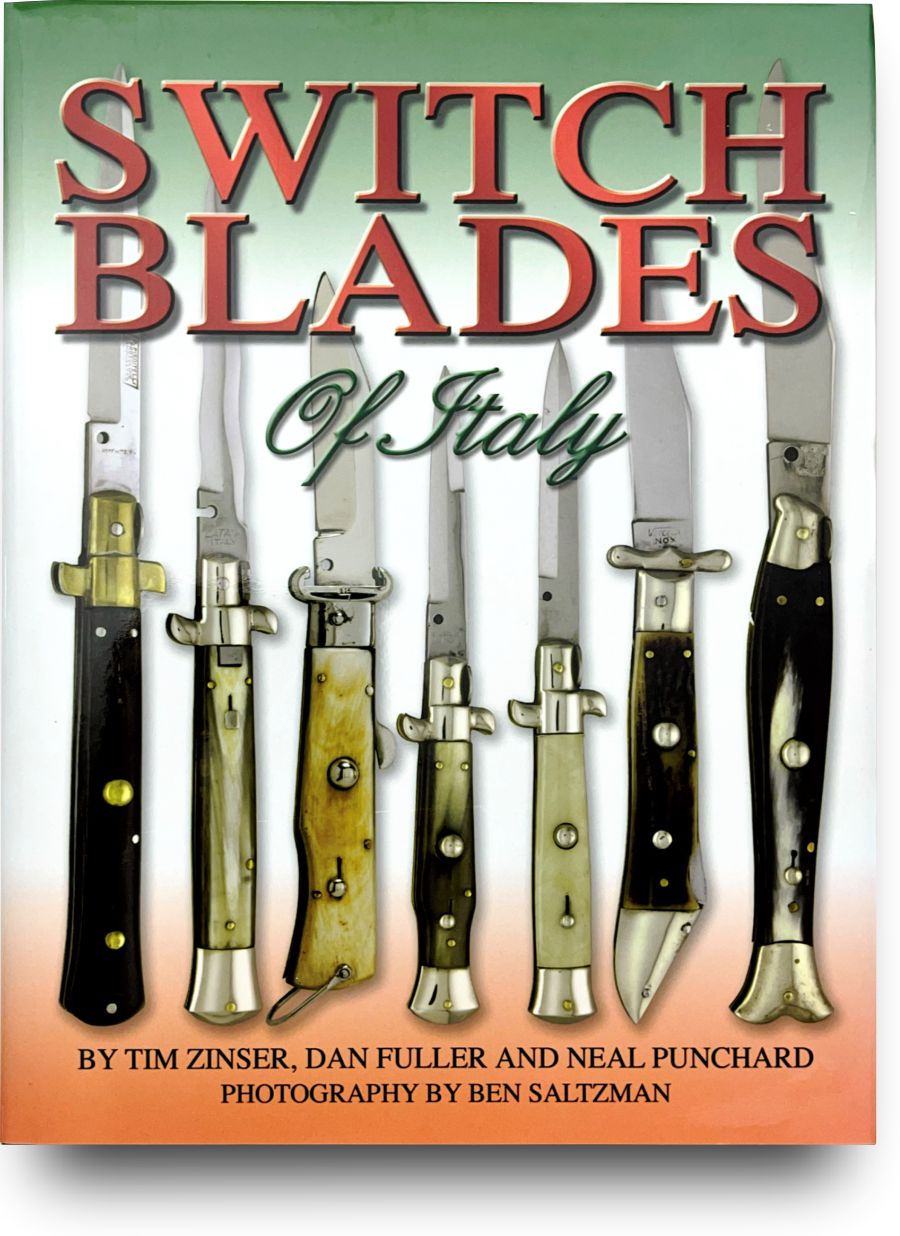This detailed book cover features a vibrant background designed to resemble the Italian flag, beginning with a green top, transitioning to a white middle, and ending with an orange-red bottom. The top showcases the bold title "Switchblades" in red uppercase letters, followed by "Of Italy" in elegant green cursive. The central focus is a vivid photograph of seven distinct switchblades, each with a unique handle ranging from Mother of Pearl, wood, ivory, black, silver, to brass, emphasizing the diverse craftsmanship of Italian knives. At the bottom, the cover credits the authors Tim Zinser, Dan Fuller, and Neil Punchard, with photography by Ben Saltzman. The book promises an in-depth exploration of the various switchblades used or available in Italy.